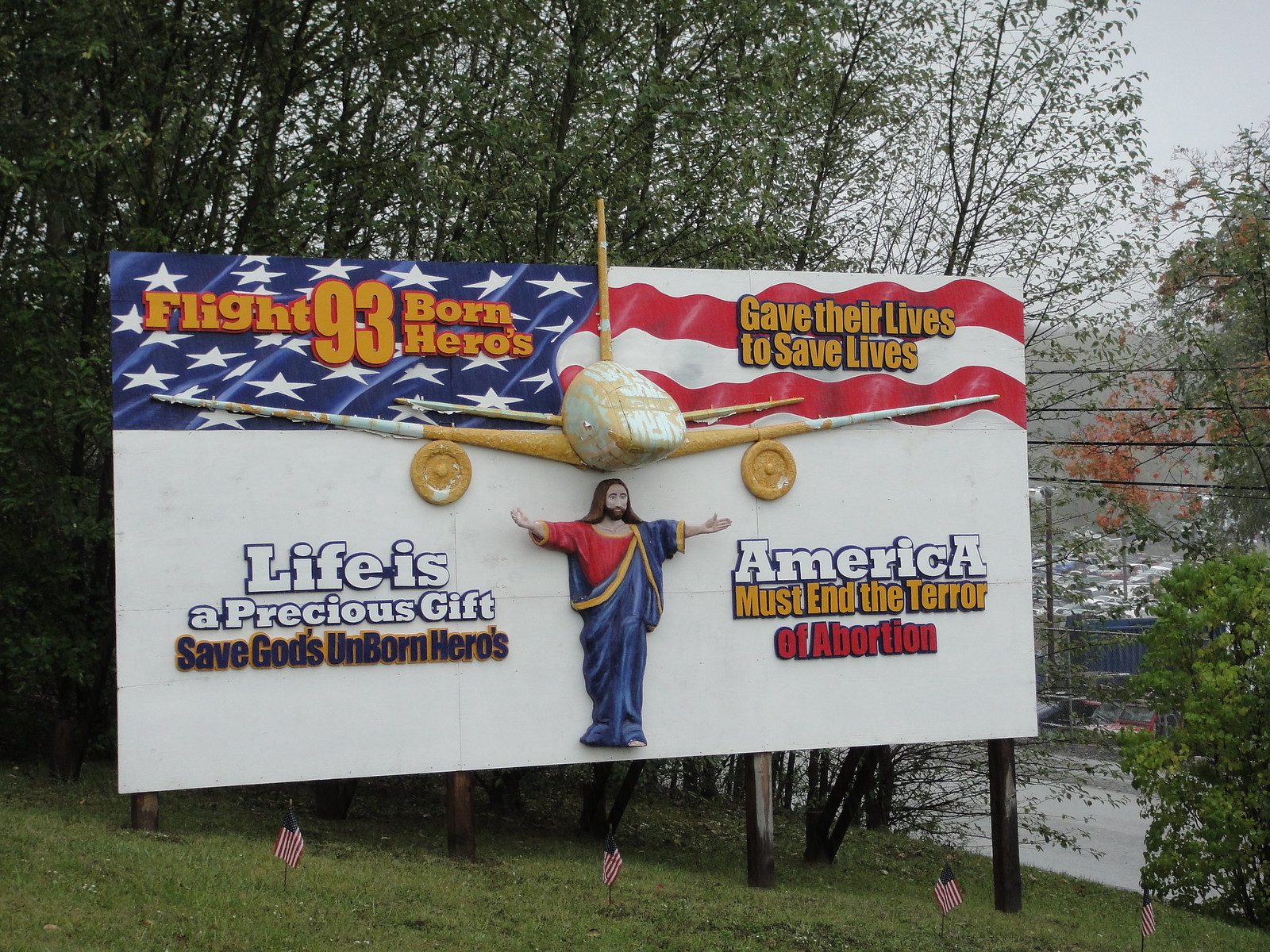This photograph captures a roadside billboard held up by four wooden poles with green trees in the background and a large car lot visible in the distance to the right. At the base of the billboard, small American flags are stuck into the green grass in a line. The billboard features a prominent American flag in the background and is filled with text and imagery. In the upper left-hand corner, the billboard reads "Flight 93, Born Heroes," while the upper right-hand corner states "Gave Their Lives to Save Lives." The centerpiece of the billboard includes a cutout of a large, yellow and white commercial jet, positioned directly above a depiction of Jesus in a blue robe with gold trim and a red tunic, his arms outstretched. Below Jesus, the text reads "Life is a Precious Gift," and continues with "Save God's Unborn Heroes" on the bottom left and "America Must End the Terror of Abortion" in bold, varied colors on the bottom right. This billboard appears to be an anti-abortion message using the valor of Flight 93 as a symbol.